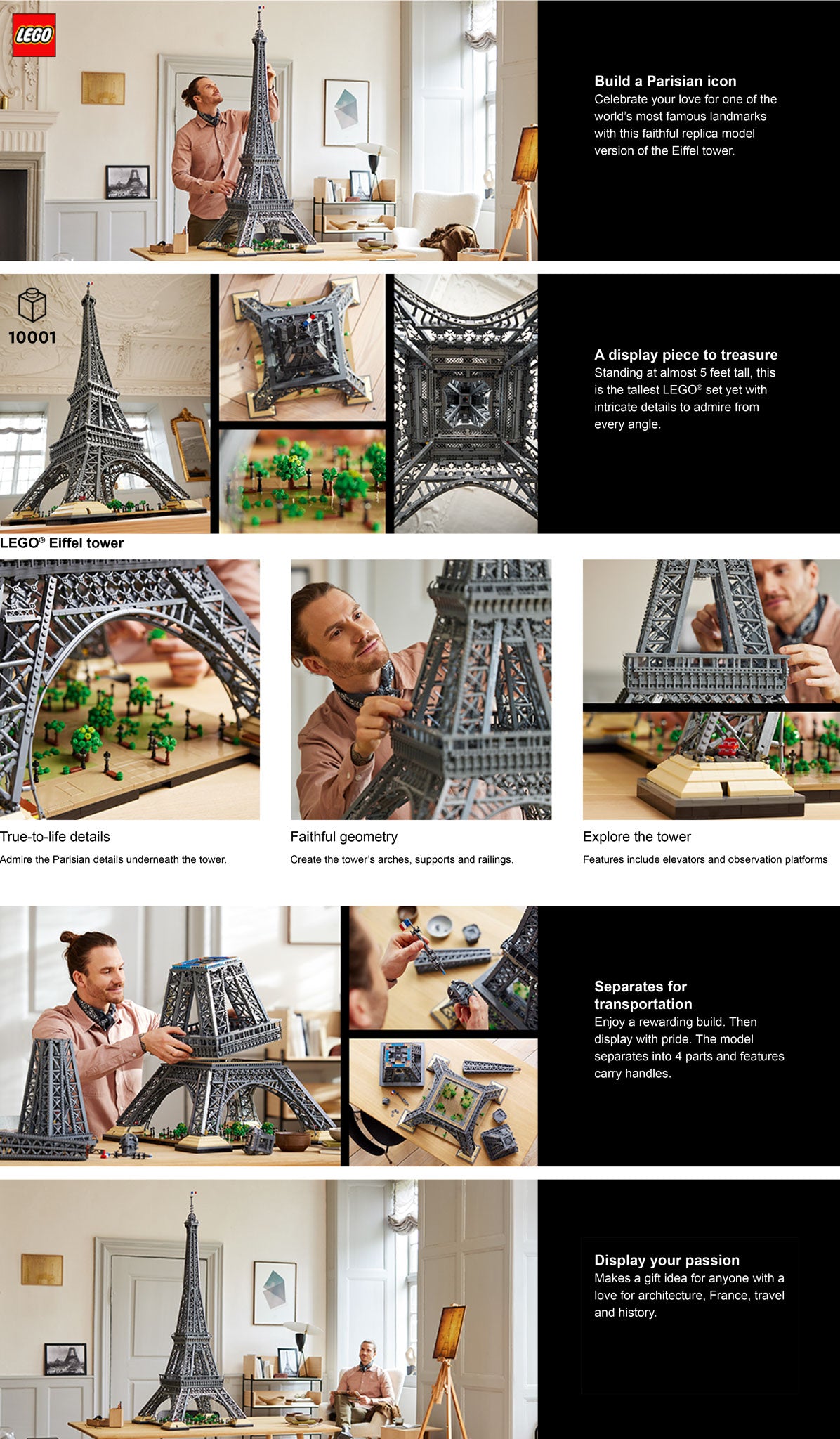This image is an advertisement for a LEGO set featuring a highly detailed replica of the Eiffel Tower. At the top left corner, the familiar LEGO emblem is displayed prominently. The advertisement comprises various pictures and text descriptions divided into multiple rows. 

The top section of the ad highlights a photograph of a man standing in front of the half-assembled Eiffel Tower model, showcasing the impressive scale as the tower extends from his waist to above his head. Alongside, there's a caption: "Build a Parisian icon. Celebrate your love for one of the world's most famous landmarks with this faithful replica model version of the Eiffel Tower."

The next row features various perspectives of the model, including an aerial view and a close-up from below, emphasizing intricate details. Text on the side reads: "A display piece to treasure. Standing at almost five feet tall, this is the tallest LEGO set yet, with intricate details to admire from every angle." Close-up images of the tiny trees at the base of the tower are also shown here.

Further down, the man is depicted actively building the tower, with captions explaining the building process: "Enjoy a rewarding build, then display with pride. The model separates into four parts." Text also highlights practical details like the separability for transportation and carry handles. Finally, the completed model is showcased with the man admiring his work. The bottom text proudly states, "Display your passion."

The advertisement combines detailed imagery of the building stages, close-ups of the model's features, and enthusiastic text to emphasize the intricacy and grandeur of the LEGO Eiffel Tower set, a perfect gift for anyone passionate about architecture, France, travel, or history.